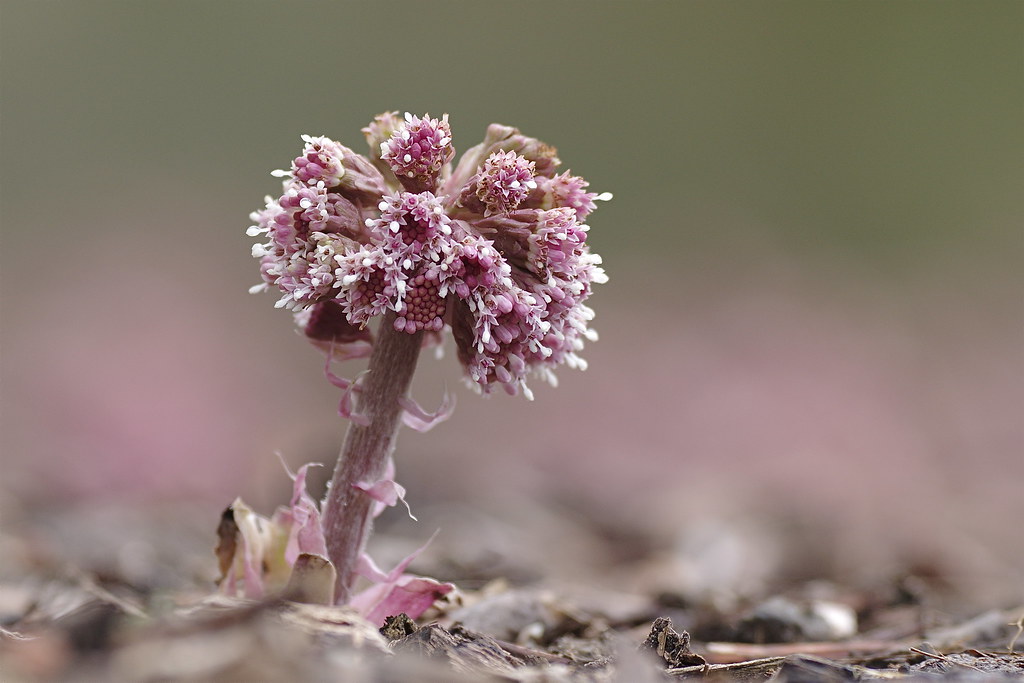This close-up photograph captures a distinctive pink flower set against a blurred background of pink and tan hues. The focal point of the image is a thick, pinkish stalk emerging straight from the ground, bypassing the traditional leafy vegetation usually associated with flowers. The stalk ends in a circular, spherical bloom composed of approximately 15-20 closed tube-like petals, which exhibit a gradient from dark pink at the center to lighter pink edges, giving the impression of a delicate sprinkling of white glitter on their tips. Surrounding the flower's base, bits of debris and fallen flower segments are scattered, alongside unrelated tan debris like twigs and dead leaves. The blurred backdrop includes hints of other foliage and vegetation, emphasizing the flower's vibrant presence and intricate details.